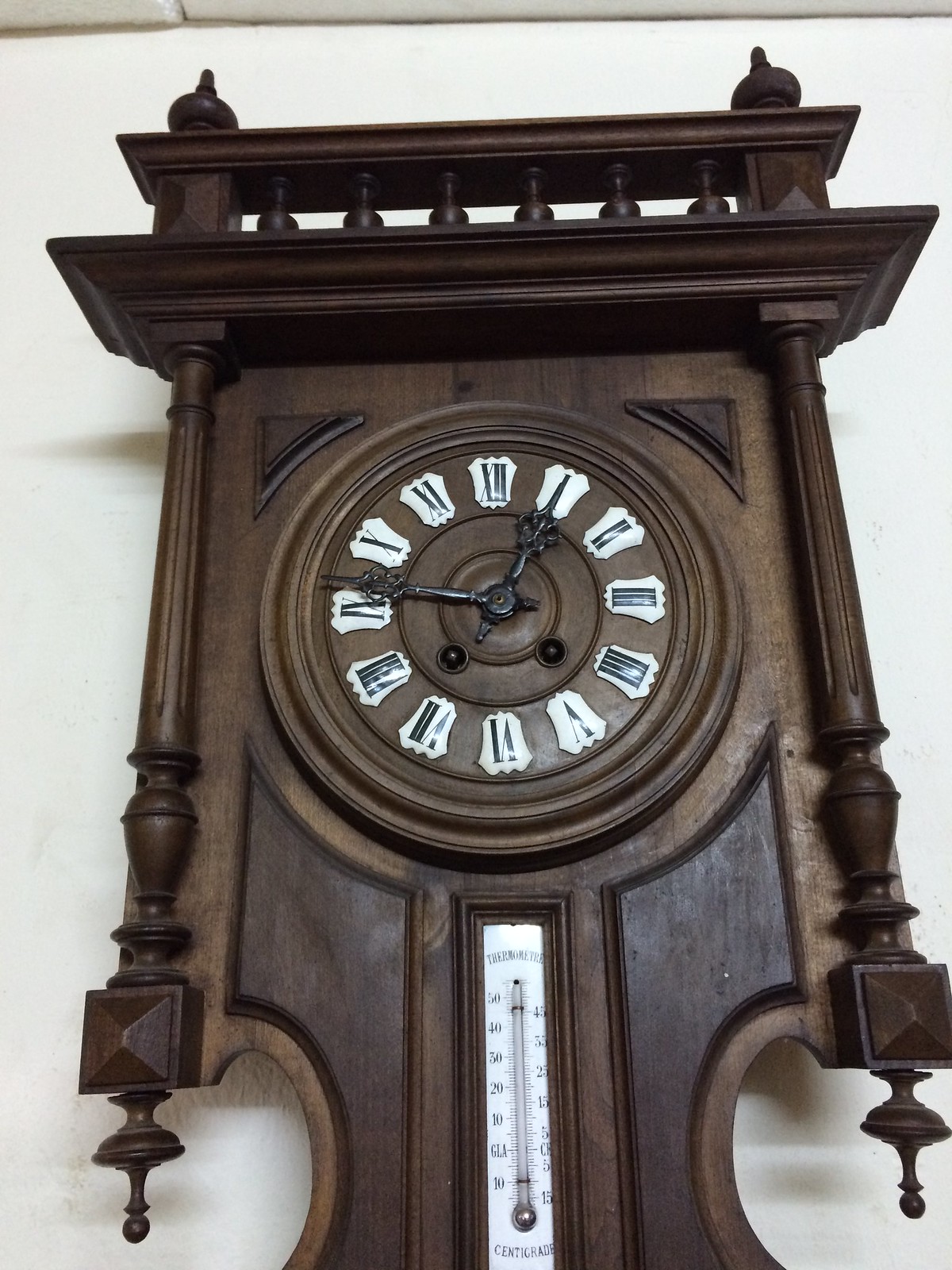A decorative wall clock is centrally positioned with a pair of small triangular designs at both the top left and top right corners. The clock face, adorned with intricate designs on the left and right sides, is framed by two posts on either side, resembling pillars. At the very bottom center, a combination of a thermostat and thermometer, showing both Celsius measurements, is embedded. The clock features Roman numerals arranged in a traditional circular layout from 1 to 12, with the minute hand resting between 1 and 2, and the hour hand positioned between 9 and 10, indicating the time. The numbers are encapsulated within a perpendicular shield-like design, adding to the ornate character of the clock.